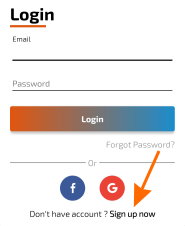This image depicts an old login page for an unspecified service or application. The layout is portrait-oriented, indicating it was likely taken from an older device. At the top, the word "login" is boldly displayed in black, underlined with an orange line. Below, there are input fields: one for an email address and another for a password. 

Further down is a login button with a gradient effect, transitioning from orange on the left to blue on the right, with a subtle brown mix in the center. Beneath the button, "Forgot password" is written in faded text, followed by the word "or" and two symbols representing Facebook and Google login options. These symbols are a blue circle with an "F" for Facebook and a red circle with a "G" for Google.

An orange arrow edit points towards the text "sign up now" extending from the "forgot password" area. The background of the login page is plain white, adding to the simplistic design.